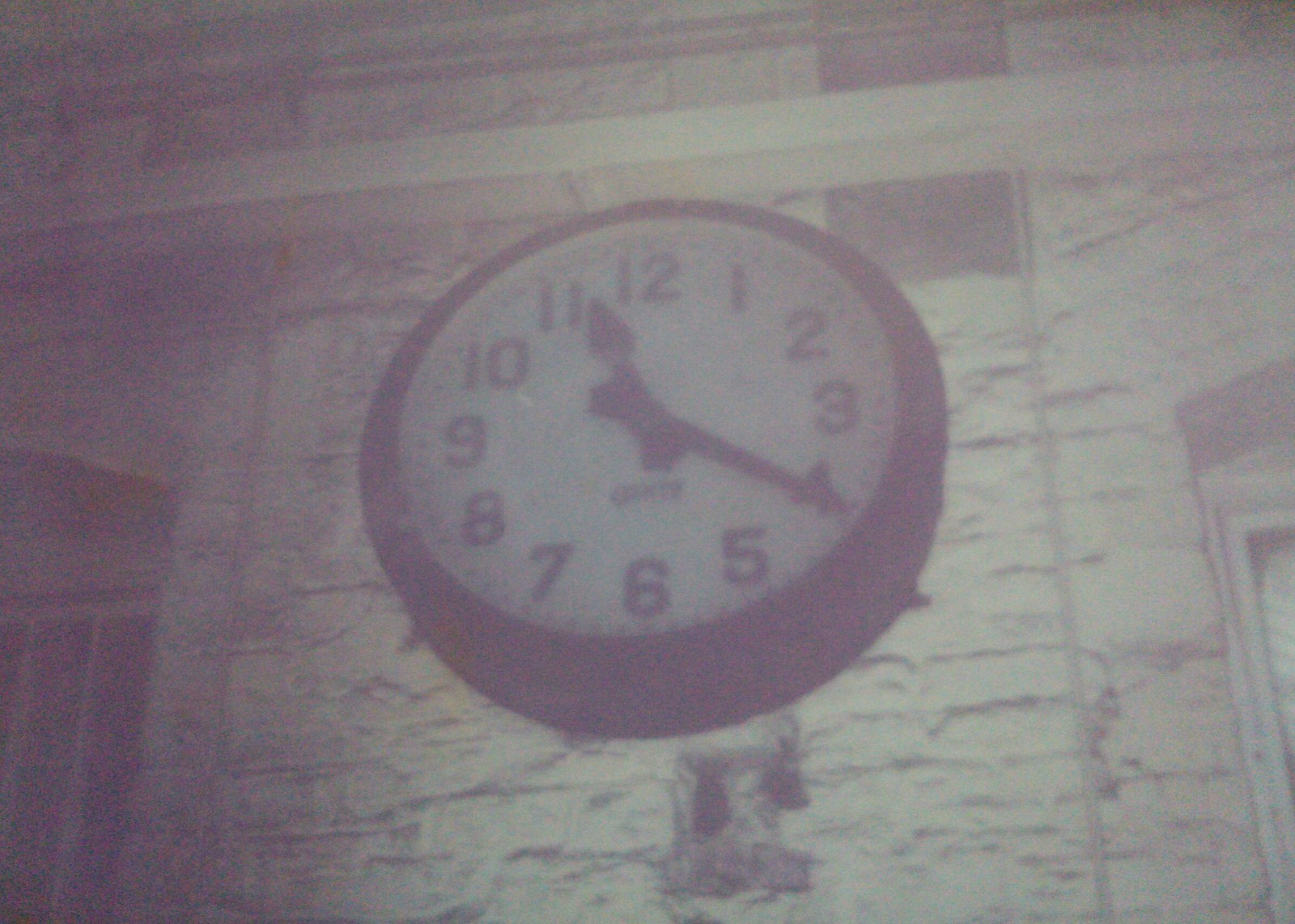The image depicts a circular wall clock with a white face, featuring large, black numbers arranged in a standard 12-hour format. The thick black hour and minute hands are positioned at approximately 11:20. The clock, adorned with an indistinct black brand name in its center, is mounted on a wall that appears to be made of stone or brick. The clock's background includes what seems like a map or a textured section with squiggly black lines. To the left of the clock is a corner of an arched window or doorway, while the right edge shows part of another arched window. The overall photograph possesses dim colors and a foggy appearance, adding to the ambiguity of the interior or exterior setting.